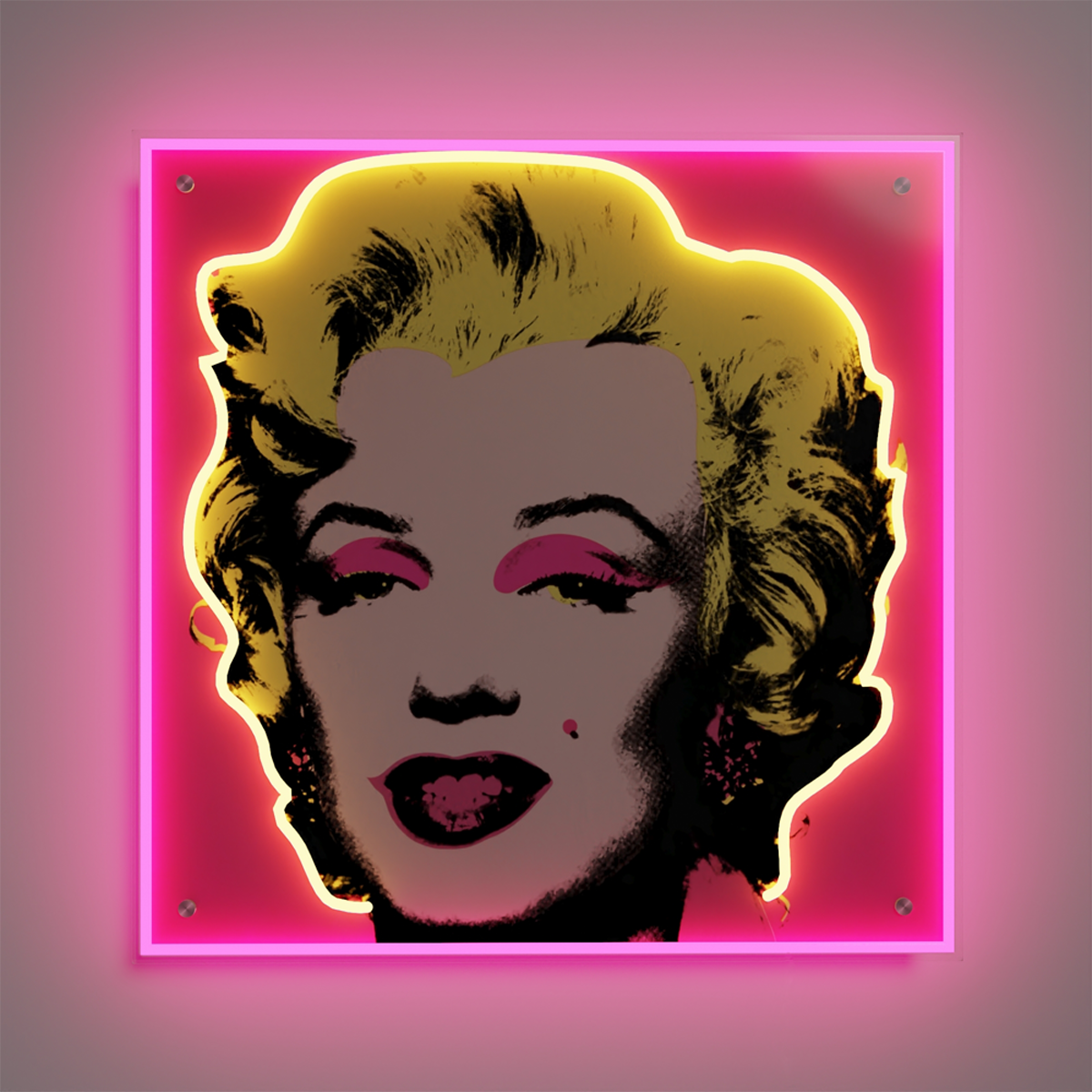The image displays a vibrant, hand-drawn, stylized portrait of Marilyn Monroe, reminiscent of Warhol's pop art style. Set within a neon-lit pink square, Marilyn's face stands out with distinct, bold colors. Her hair, rendered in a rich, curly yellow halo, is accentuated by a whitish-yellow neon strip adding a vibrant glow. Marilyn's face is predominantly white, with high-arched dark eyebrows. Her eyes, partially closed in a lazy gaze, are highlighted by yellow irises and pink eyeshadow lids. Underneath, yellow-tinted eye makeup complements her expressive look. The lower profile of her nose is visible, leading to her signature pink lips, painted in a slightly smirking expression. This striking image is further framed by a gradient from dark gray to light pink, enhancing the intense illumination and modern aesthetic of the overall portrait.